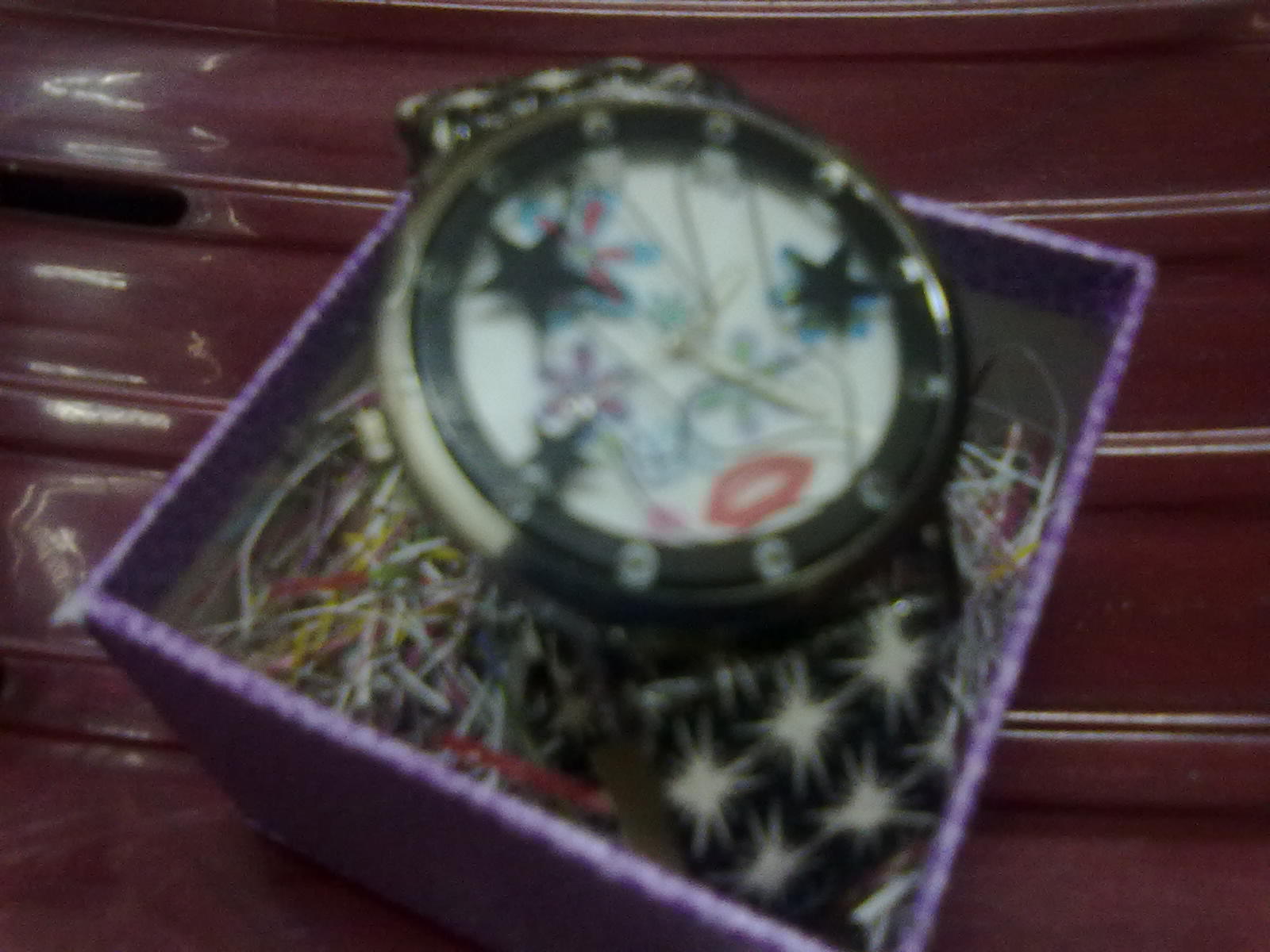The image depicts a small, vibrant purple box filled with multicolored paper shreds, evocative of Easter basket filler or present stuffing. The paper strands come in an array of colors: yellow, red, white, blue, and purple, creating a lively and festive backdrop. Resting atop this colorful bed is a watch, characterized by a black strap adorned with white luminous accents. The watch face itself is white, featuring an intricate design that showcases a hand making a peace sign, embellished with hues of red, blue, and purple, along with star motifs. Additionally, black stars are intricately placed on the top of the watch. The entire scene is set against a red, ribbed surface that appears to be made of either plastic or metal, adding an extra layer of texture to the composition.